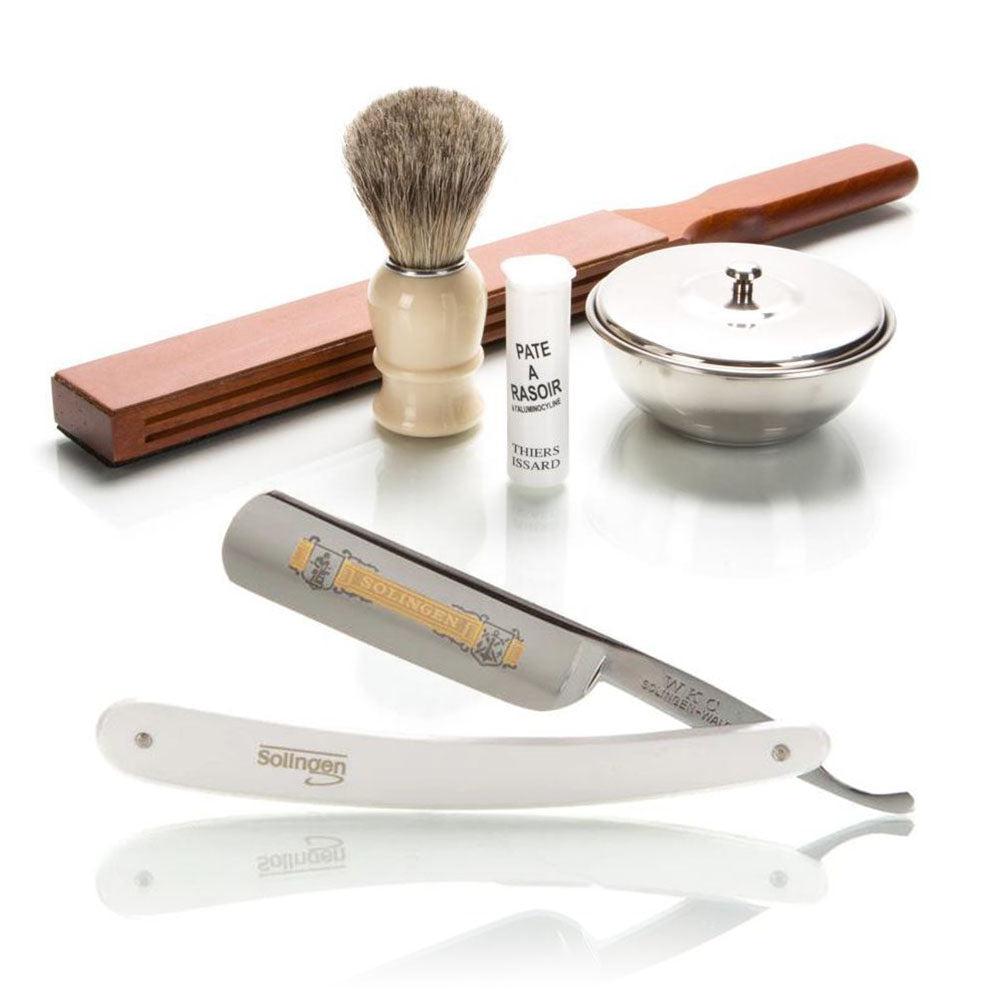This image depicts a classic men's shaving kit displayed against a white background. Central to the picture is an old-style straight razor with a white handle and silver blade, folded safely within its sheath. Behind the razor is a wooden strop for honing the blade. Adjacent to this, there's a traditional shaving brush, featuring a white wooden handle and fine bristles that transition from tan at the base to black at the tips. A stainless steel bowl with a lid, possibly used for mixing shaving cream, is visible, next to a white tube labeled "Paté à Rassor." The collection of these vintage grooming tools highlights a timeless approach to male grooming.